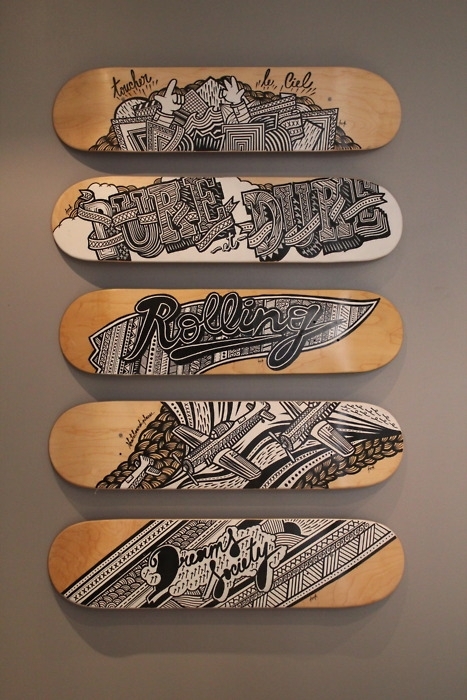This image features a striking arrangement of five highly decorative skateboards displayed horizontally against a uniform grayish-brown wall. These wooden skateboards are devoid of trucks and wheels, serving as artistic pieces rather than functional sports equipment. Each skateboard showcases intricate black-and-white designs, unified by a graffiti-like, comic-book aesthetic that evokes a sense of decorative intricacy. 

The top skateboard commands attention with its composition of several white hands emerging from geometric shapes and patterned squares, accompanied by the text "Toucher Le Ciel," giving a trippy, busy visual effect. The one immediately below it flaunts the phrase "Pure Dure" in ornate, patterned letters, intertwined with a decorative ribbon, set against a cloudy backdrop on the wooden canvas. 

Positioned centrally, the third skateboard reads "Rolling" in a cursive script reminiscent of a baseball team's logo, accentuated by a complex patterned shape that highlights the text. The fourth skateboard down features two planes soaring over an intricate, potentially bird's-eye representation of a freeway, enhanced by further geometric patterns and a braided texture that might symbolize smoke or motion. 

Finally, the bottom skateboard is adorned with the phrase "Dream Society" in filled-in cursive letters, set against a white cloudy background and surrounded by various dense patterns, forming a cohesive yet richly detailed design. Shadows cast by the skateboards and slight variations in lighting accentuate the artwork, lending depth and dynamism to the display.